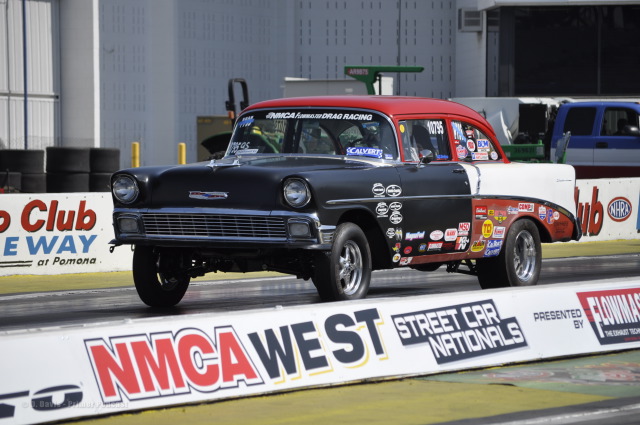The image showcases an old-style drag racing car positioned on a slightly wet track, captured in broad daylight. The car features a distinctive color scheme with a black front hood and doors, a red roof, a white trunk, and a red lower fender at the back. The vehicle is adorned with a variety of colorful sponsor stickers prominently displayed on its side. Its design includes square-shaped bodywork coupled with chrome bumpers. The car is equipped with star-shaped wheels, and the headlights are not illuminated. Surrounding the track, there are white banner borders with red, blue, and black lettering. A visible barrier right in front reads, "NMCA West Street Car Nationals presented by Flowmaster." The windshield has some text that suggests it pertains to drag racing, and in the background, stacks of tires can be seen, indicating a typical racing environment.